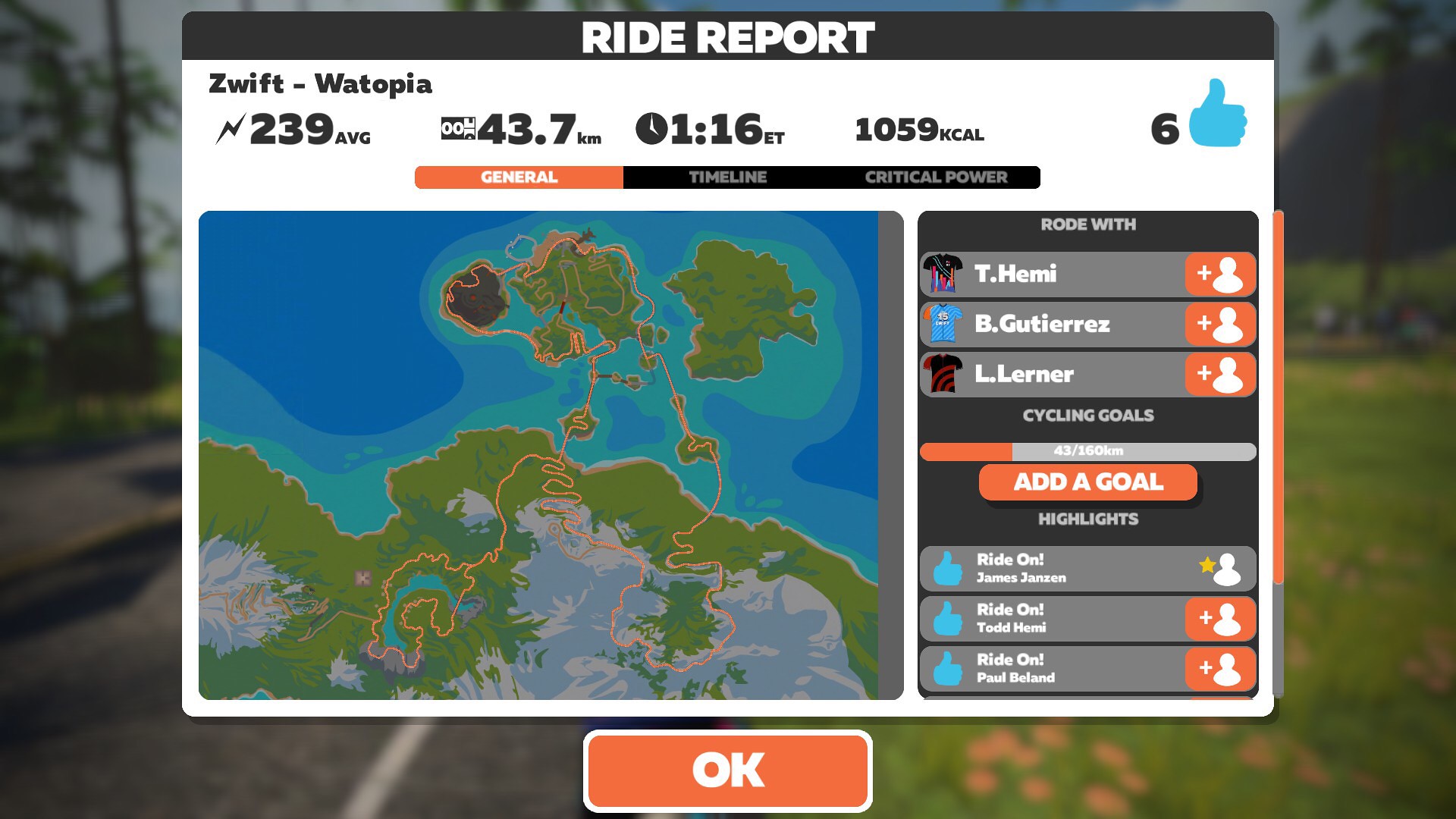This image is a detailed ride report for a Zwift cycling session in the virtual world of Watopia. At the top left, it reads "Ride Report Zwift - Watopia" with a graphic of a lightning bolt next to the average power output of 239 watts. Below, it shows that the ride covered a distance of 43.7 km in an estimated time of 1 hour and 16 minutes, burning 1059 kilocalories. The central part of the image features a map, with blue indicating water and green for land, crisscrossed by yellow squiggle lines representing the cycling route taken. 

On the right side, there is a section labeled "Road with" that lists names such as T. Hemi, B. Gutierrez, and L. Learner, each accompanied by a graphic of a cycling jersey and a silhouette of a head and shoulders. Below these names, the document mentions cycling goals, one of which reads "45/43 out of 160 km." Additionally, there's an orange box prompting users to "Add a Goal," with highlighted "Right On" comments from other users, including James Jensen, Todd Hemi, and Paul Beland, each marked with a thumbs-up graphic. This comprehensive ride report overlays the screen of the virtual cycling environment, combining detailed statistics, social interactions, and visual route mapping.